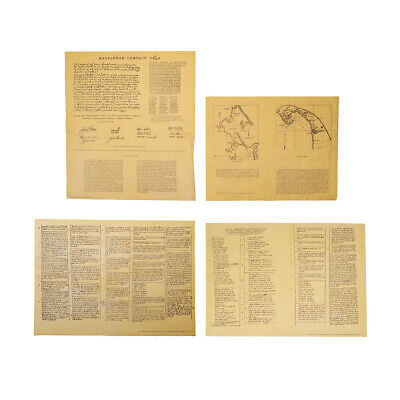The image depicts four aged, possibly oxidized pages set against a white background, appearing as though they are from an old book. The pages are arranged with two on the top and two on the bottom, each exhibiting varying shades of tan to light brown, suggesting they are quite old. The top left page has an orangey parchment-like appearance and features almost signature-like markings in the middle, while the top right page displays two diagrams that resemble maps or other land-like imagery. The bottom two pages are lighter in color, identical in size, and filled with tiny, repetitive paragraphs of black text. Due to the blurriness and distance of the photo, the specific content is indecipherable, but the overall impression is of ancient, weathered documents.